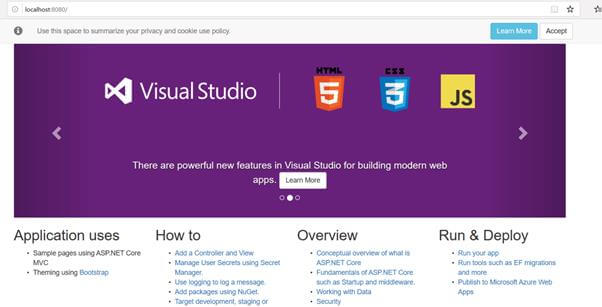Here is a detailed and cleaned-up caption for the described image:

---

The screenshot displays a webpage featuring a white background with a minimalistic design. At the top, there is a website address section, accompanied by an icon depicting a white eye encased in a gray circle. Below this, the page contains a text area inviting users to "Use this space to summarize your privacy and cookie use policy." Adjacent to this text, there are two interactive buttons: a blue rectangular button labeled "Learn More," and a white rectangular button labeled "Accept."

Further down, a prominent purple rectangle showcases information about Visual Studio, highlighting its powerful new features for building modern web apps. This section emphasizes key technologies with icons: a "5" for HTML, a "3" for CSS, and a "JS" for JavaScript. 

Additionally, the page includes another white rectangular button labeled "Learn More."

Towards the bottom of the screenshot, there are three navigation dots, with the middle one shaded white, indicating the current view. The content in this section elaborates on application uses with information, categorized into three main areas, each highlighted in blue:
1. "How To" - Featuring a list of actionable information.
2. "Overview" - Offering a summarized list of details.
3. "Run and Deploy" - Detailing the steps for running and deploying apps, including references to running your app, migrations, and other processes beginning with "M."

---

This comprehensive caption provides a structured and detailed description of the image's contents.